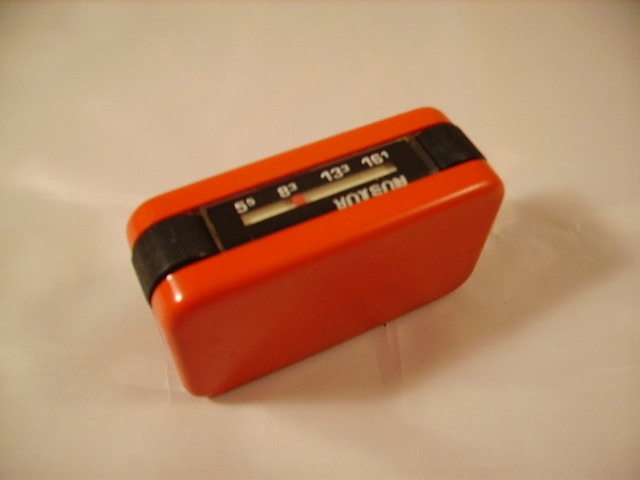A shiny, smooth, small rectangular object made of orange plastic rests on a white surface. Centered on the orange object is a black stripe, adorned with four sets of numbers: \(5^5\), \(8^3\), \(13^3\), and \(16^1\), each representing different values. A tiny red pointer, situated within an open spot on the black stripe, is currently aligned with \(8^3\). Below these numerical values, there is white text that seems to form a logo, although the precise wording is unclear. The object reflects the light, making its glossy surface apparent.